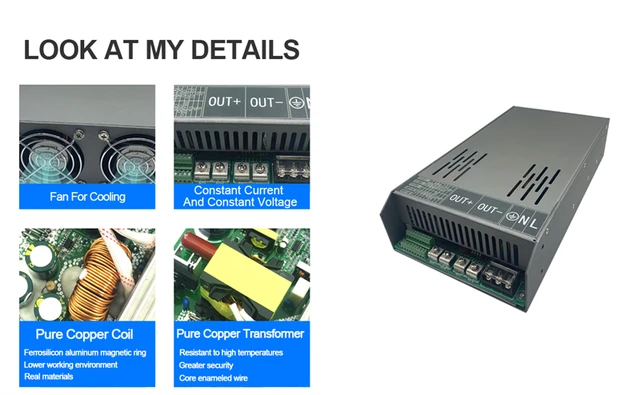The image showcases an electronic device, specifically a gray rectangular box with distinct markings and connectors. On the right side of the image, the device is labeled with "Out +" and "Out -", alongside "End" and "L" symbols, indicating various electrical outputs and connection points. The device features ventilation slits on the top and bottom to ensure proper cooling. The left-hand side of the image includes detailed annotations under the heading "Look at my details." Here, four informational squares provide further insights: the top left square highlights a "Fan for cooling" with an accompanying image of the fan; the top right square emphasizes "Constant current and constant voltage" with a photo illustrating the relevant buttons; the bottom left square describes a "Pure copper coil" with "ferrosilicon aluminum magnetic ring" and an image of the components; the bottom right square details a "Pure copper transformer" noted for its resistance to high temperatures and superior security, supported by a visual of the copper transformer. This comprehensive depiction offers a clear understanding of the various features and components of the electronic device.